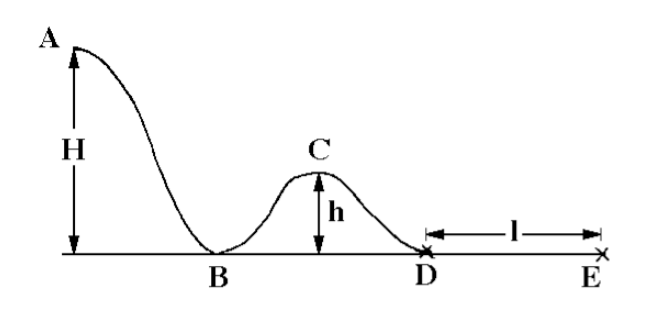This image depicts a detailed digital graph, likely created using pixel art, set against a white background. The graph aims to demonstrate a sequence of data points and annotations along both vertical and horizontal axes. 

Starting from the left-hand side, there is a vertical arrow with an "H" at its center. At the top of this arrow, labeled "A," a curved line descends approximately a quarter way down the graph to point "B." The line then moves upward slightly to point "C." The graph includes a second vertical arrow beneath "C," marked with a lowercase "h." The line dips down again to about three-quarters along the length of the graph, reaching point "D." From point "D," a horizontal arrow extends to the right, culminating at an "X" that marks the end of the line, labeled "E."